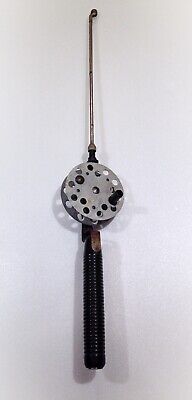The image is a highly detailed color photograph of an object that resembles an ancient or abstract fishing rod, set against a white or beige backdrop. At the bottom, the rod features a short, black, ribbed, and semi-reflective handle with a grip in the middle. Extending from this handle, there is a metallic circular reel, filled with numerous cutouts or smaller circles. Emerging from one of these cutouts is a black rod, and atop the reel, a small metal rod protrudes through the handle, ending in a hook-like figure with a ball tip rather than a sharp point. This entire structure casts a distinct shadow on the white backdrop. The photograph focuses solely on this singular, intricate object without any accompanying text, people, animals, or other mechanical items.